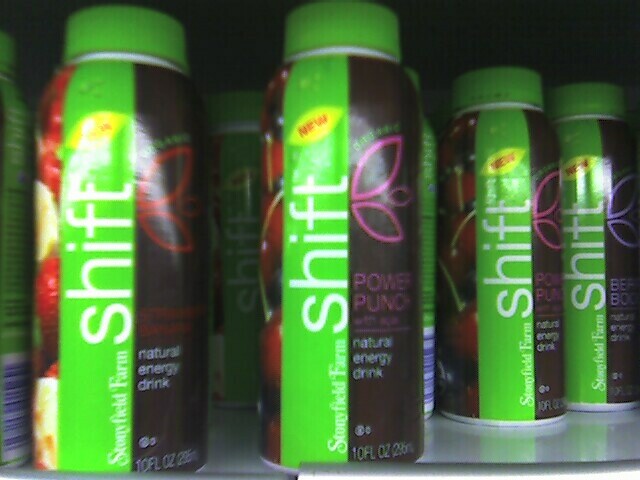The image displays four bottles of an energy drink brand called "Shift." Each bottle features a prominent green stripe down the center with the brand name "Shift" printed vertically in green. The green stripe is flanked by colorful panels on either side, each showcasing different fruit images and flavor names, although some are too blurry to read clearly. The bottles have noticeable green caps and small yellow labels that indicate "new." 

The first bottle on the left features a red and yellow design with an outline of leaves in red and black. It prominently displays the phrase "natural energy drink" in white and lists "ten fluid ounces" below. The second bottle follows a similar design but with purple outline leaves and writing in purple, suggesting a different flavor. 

Each bottle seems to depict images of various fruits: the nearest one shows cherries, indicating a "Power Punch" flavor, while another appears to have strawberries and bananas. One more bottle is labeled "Berry Boost," though the fruit images on this one are not clearly visible. The overall aesthetic includes a mix of red, yellow, black, and green, with the bottles aligned in a row.